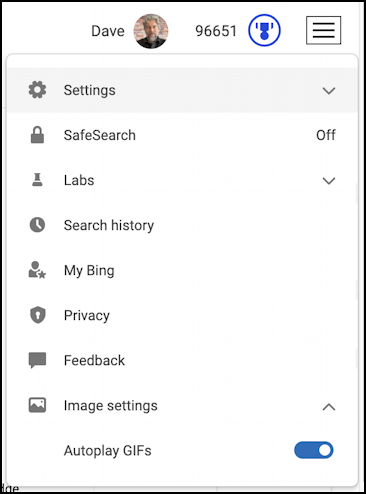Detailed Caption:

This image depicts a section of a website featuring a profile picture of a man named Dave. Dave is a Caucasian male dressed in a black suit. Adjacent to his profile picture, the number "96651" is displayed, accompanied by a blue icon. The icon resembles a box with a circle beneath it and two lines extending from each side.

Below this section, there is a gray box with horizontal lines, which seems to compartmentalize different settings options. The visible options include "Settings," "Safe Search," and "Labs," each accompanied by drop-down menus. To the right of "Safe Search," the text indicates that it is turned off. Other options listed are "Search History," "My Bing," "Privacy," "Feedback," and "Image Settings," the last of which features an upward-pointing arrow next to it.

Further down, the option "Autoplay GIFs" is presented with a blue slider positioned to the right, likely indicating it is enabled. The settings options are confined within a thinly outlined gray box, and the entire website appears to have a black outline. Outside the settings box on the left side, barely discernible letters, possibly "L-O-E," are visible.